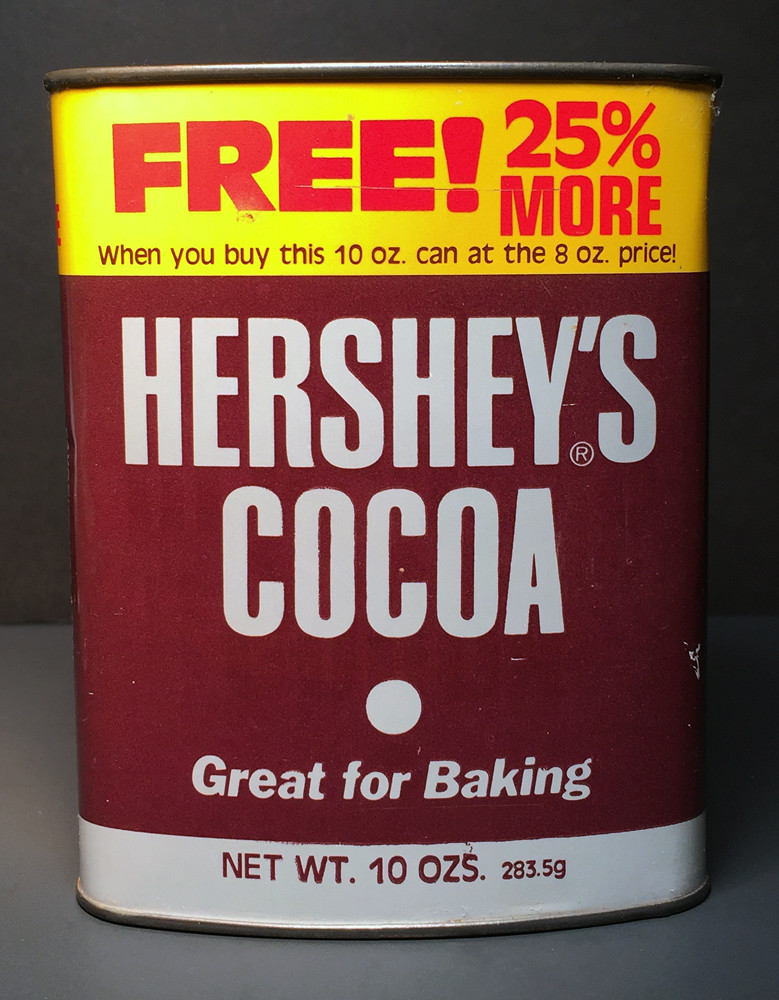The image features a vintage Hershey's Cocoa canister, reminiscent of an 80s design. The rectangular container is predominantly chocolate brown, with a distinct yellow band at the top quarter of the label. In bold red lettering within this yellow section, it proclaims "FREE! 25% MORE," followed by brown text stating, "when you buy this 10 ounce can at the 8 ounce price!" Below the yellow band, the central portion of the label is dominated by the Hershey's Cocoa branding in large, prominent silver letters, accompanied by the slogan "Great for baking." The bottom sixth of the label has a silver band with brown text, specifying the net weight as "10 OZ" (283.5 grams). The can is positioned on a gray table against a black backdrop.